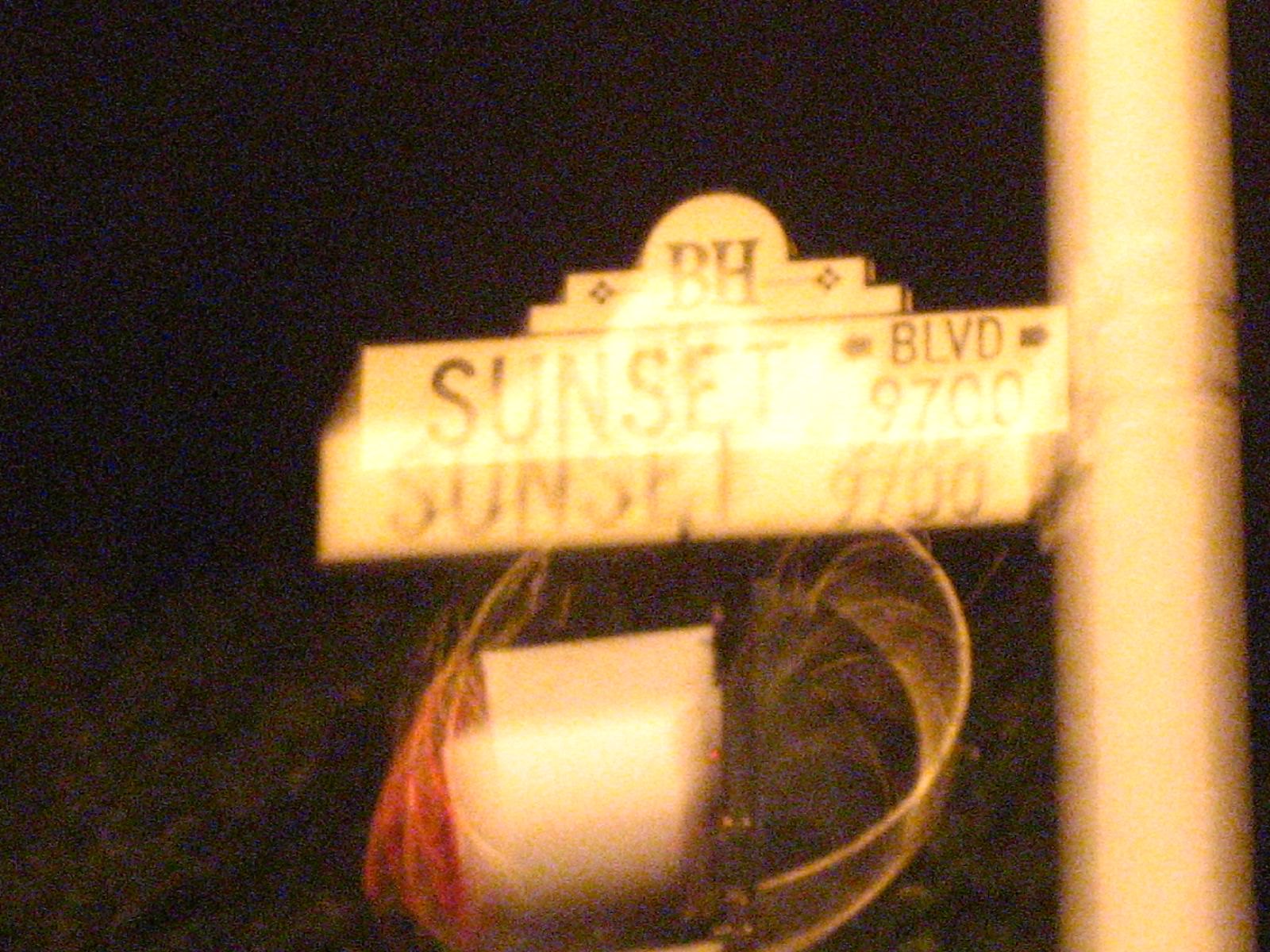The photograph depicts a street sign mounted on a white, slightly gray cylinder post, likely situated by the side of a street. The overall color scheme of the image features predominantly black and green hues. In the background, green foliage is visible at the bottom, blending into the dark, night sky above, which casts a hazy, nocturnal ambiance over the scene. 

The post supports a white, rectangular street sign with an elegant, vintage design reminiscent of an old theater marquee. The sign prominently displays "BH," followed by "Sunset Boulevard BLVD 9700." Due to the nighttime setting and image blur, the street sign's text appears to repeat below it, creating a ghostly, double-vision effect. Additionally, two concentric circles of yellow light are visible underneath the sign, adding a surreal touch to the night scene.